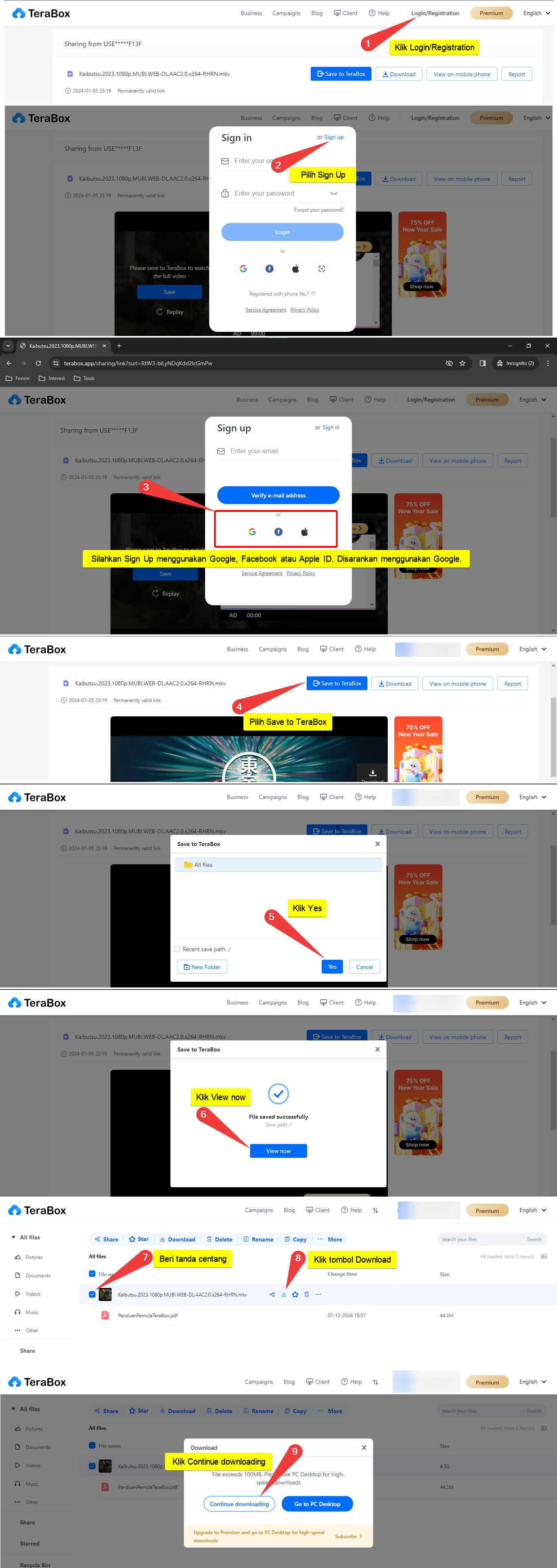This image features a computer screen segmented into multiple distinct sections. At the top, there is a noticeable white border, followed by two prominent pop-up windows overlaying a desktop interface. Each pop-up window has a gray background with interactive elements. 

The first pop-up contains a small white square positioned centrally with a thin orange line inside. Below this square, a segment is highlighted, leading to a blue-bordered button at the bottom, implying interactivity.

Similarly, the second pop-up window below mirrors the structure of the first, featuring a white square with an orange boxed area to the left of a small line. Beneath it, a yellow-highlighted segment stands out. 

As the screen drifts downward, various visual cues in red direct the user's attention to specific areas. Notable among these is a red indicator pointing towards a blue button in the section that follows. 

The screen continues in this instructional manner to the bottom, using red lines and highlighted sections to guide the user through a sequence of steps, presumably to navigate or complete a process on the website.